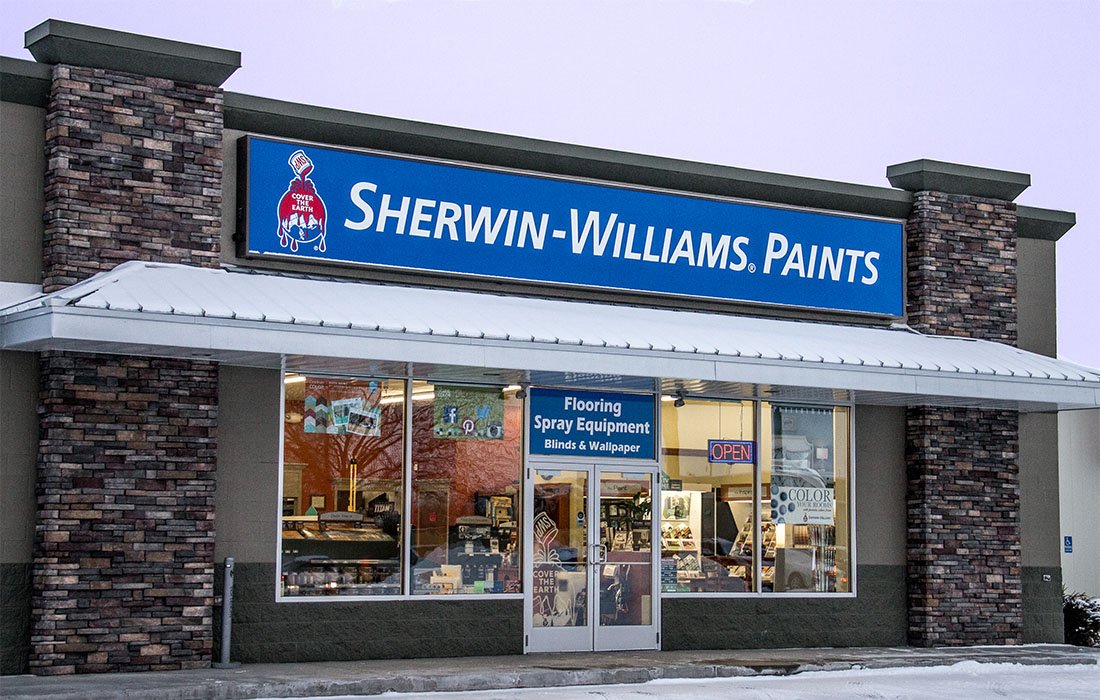This color photograph captures a Sherwin-Williams Paints store from a slight diagonal angle. The backdrop presents a very gray and overcast sky, devoid of any visible clouds. The store features gray brick pillars on both its left and right sides, while a white awning spans across the storefront. Dominating the top of the building is a prominent blue rectangular sign, displaying "Sherwin-Williams Paints" in all capital, white letters. Adjacent to "Sherwin" is the well-known Sherwin-Williams icon: a globe being drenched in red paint from a tilted paint can above it, accompanied by the phrase "Cover the Earth" and dripping red paint. 

The photo also reveals the store's glass windows, which reflect the silhouettes of nearby trees. The window displays various advertisements, with a notable "OPEN" sign on the right side, suspended by two cables. This sign is a black rectangle, bordered by blue neon and featuring the word "OPEN" in bright red neon letters. An additional sign above the double front doors lists "Flooring, Spray Equipment, Blinds, and Wallpaper." Each front door has a silver door handle. The scene includes a gray sidewalk in front of the store, leading to a parking lot that is visibly covered with a layer of snow.